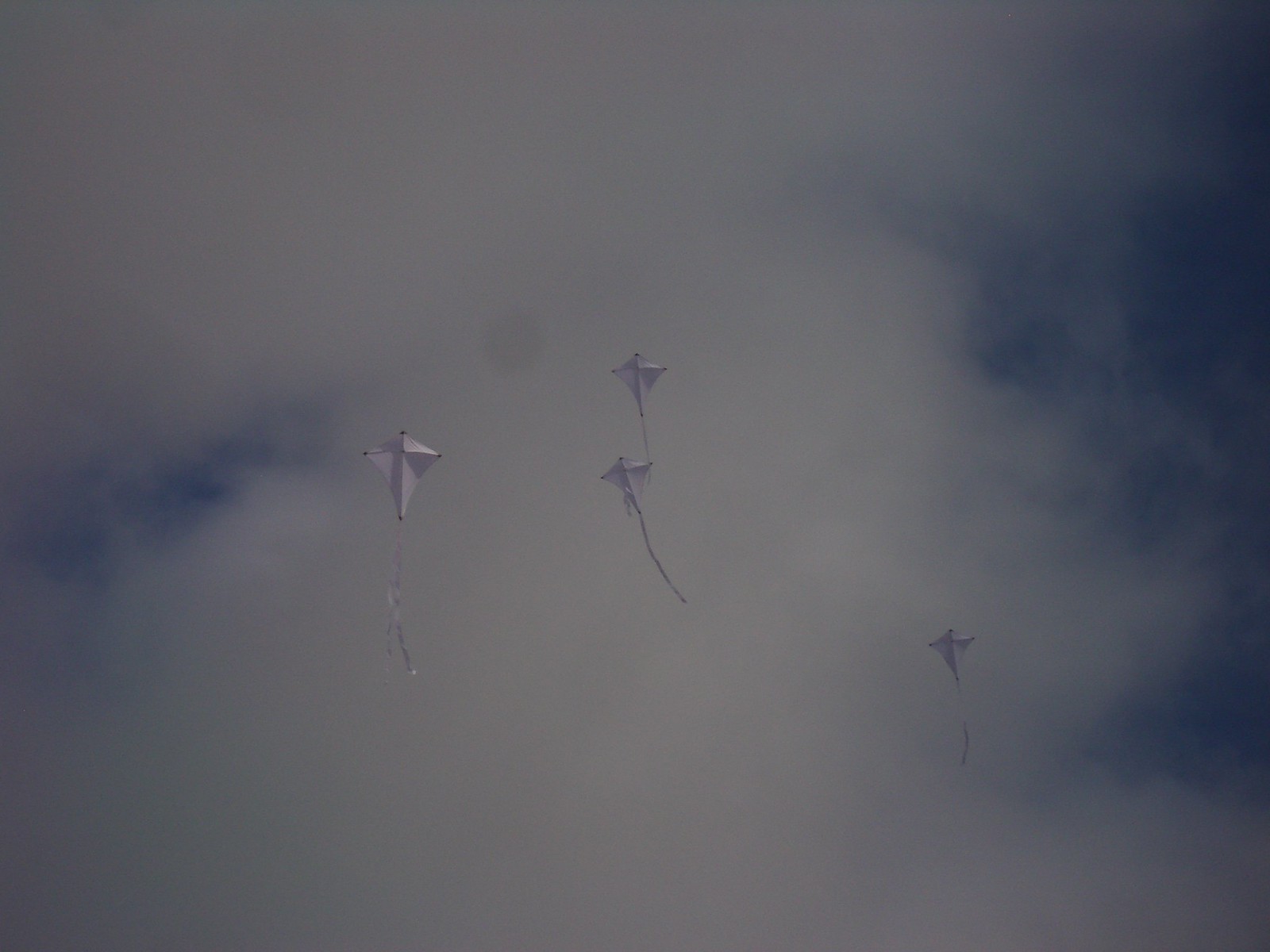The image captures a serene scene of four white kites soaring against a cloudy, blue sky. These kites, all of a similar muted white shade, are simple in design, shaped like diamonds with white material stretched over their frames. Each kite features a singular white tail trailing beneath it. The sky is dominated by thick, billowy clouds with only slivers of darker blue sky peeking through in some areas, particularly in the left center and right side. Three of the kites are grouped closer together towards the left side of the image, with two almost stacked one above the other in the center. The fourth kite is lower in the sky, near the bottom right, almost appearing to float behind the cloud cover. Despite the image not being very sharp, it conveys what was likely a beautiful day, albeit largely overcast. There are no text elements within the image.